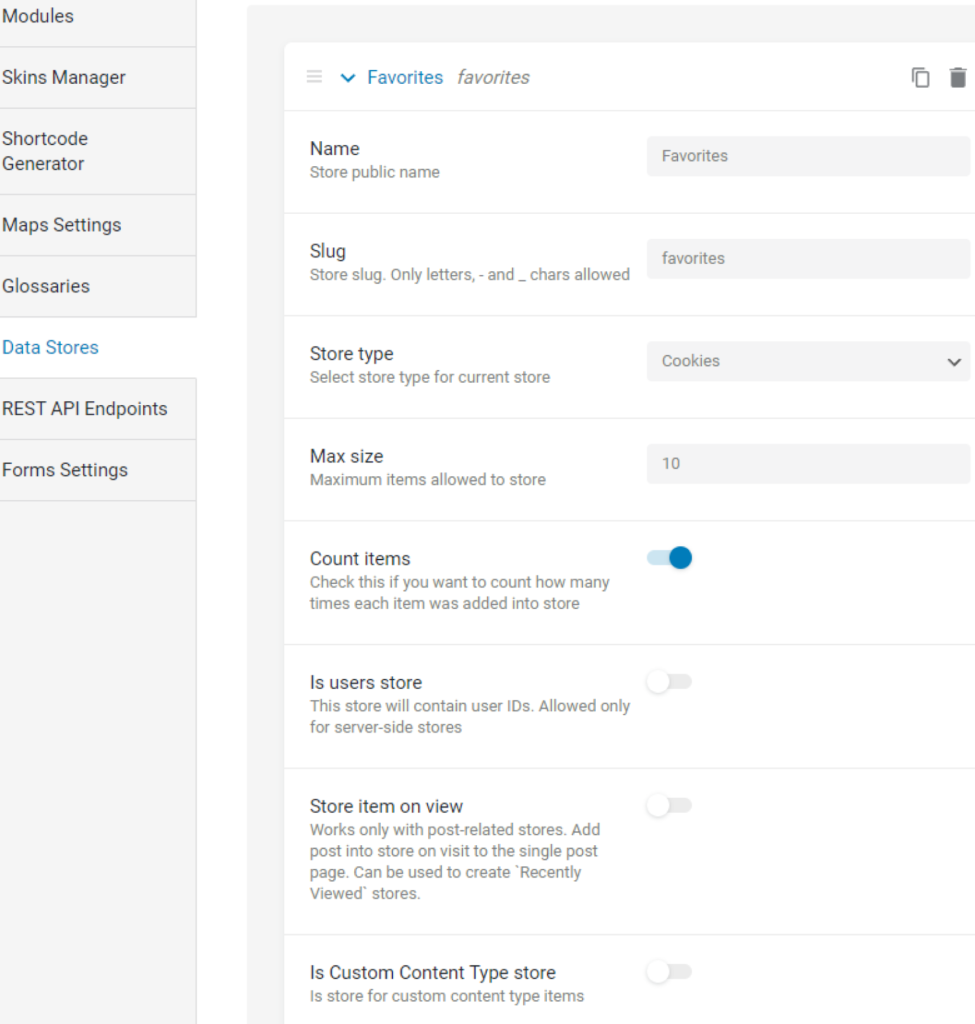This image depicts a settings page for an unnamed app. The interface is divided into two primary sections. On the left side, there is a vertical menu showcasing various categories, listed in the following order from top to bottom: 

- Modules
- Skins Manager
- Short Code Generator
- Maps Settings
- Glossaries
- Data Stores (highlighted)
- REST API Endpoints
- Forms Settings

The right side displays the main content area with the "Data Stores" section selected. Here, a dropdown menu labeled "Favorites" is visible at the top. Below this menu, various configurable fields and toggles are presented:

1. **Name:**
   - Label: "Store Public Name"
   - Text Field: "favorites"

2. **Store Slug:**
   - Instruction: "Only letters and underscore characters allowed."
   - Text Field: "favorites" (in lowercase)

3. **Store Type:**
   - Instruction: "Select store type for current store."
   - Dropdown Menu: "Cookies"

4. **Max Size:**
   - Instruction: "Maximum items allowed to store."
   - Text Field: "10"

5. **Count Items:**
   - Instruction: "Check this if you want to count how many times each item was added into store."
   - Toggle: Set to "On" (blue)

6. **User's Store:**
   - Instruction: "This store will contain user IDs allowed only for server-side stores."
   - Toggle: Set to "Off" (grayed out)

7. **Store Item on View:**
   - Instruction: "Works only with post-related stores. Add post into store on visit to this single post page. Can be used to create recently viewed stores."
   - Toggle: Set to "Off" (grayed out)

8. **Is Custom Content Type Store:**
   - Instruction: "Is store for custom content type items."
   - Toggle: Set to "Off" (grayed out)